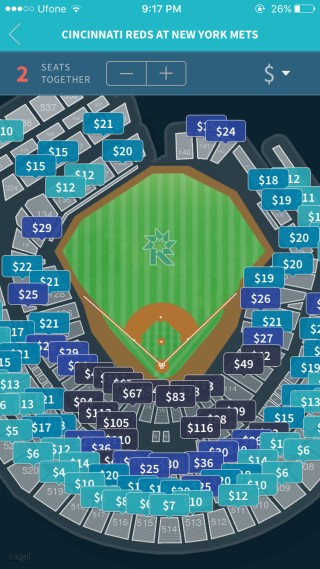The image depicts a webpage displayed on a smartphone. The header of the webpage is light blue and features white text that reads "C.I.N. Sinati," followed by "right at New York meets." Below this, in red and white text, it says "Two Seeds Together," with the word "Two" in red and "Seeds Together" in white. 

To the right of this text, there are plus and minus symbols as well as a dollar sign. The main body of the webpage displays a football field in the center, which is green with a stylized, slightly blue 'R' at its center, accompanied by brown and white lines marking the field. Surrounding the 'R' is a spiral containing various prices.

The prices are listed in different colors based on their values. Prices less than $20 are light blue, including $24, $36, $27, $25, and $29. Prices that are slightly higher, above $25, are indicated in dark blue and include $67, $83, $105, $116, and $49. The remaining prices, which are above these amounts, are shown in black. Each price is carefully placed along the spiral encircling the field, creating an organized yet visually engaging presentation.